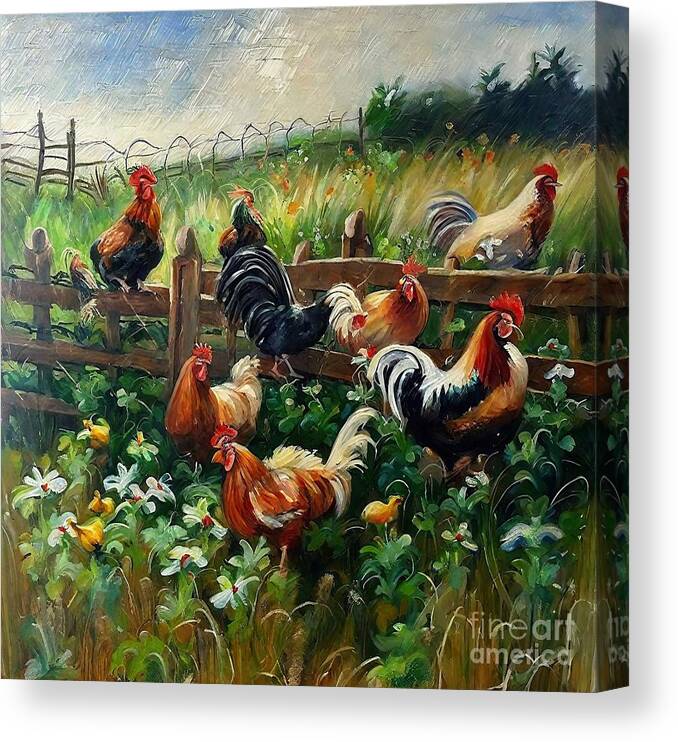The painting depicts a vibrant farm scene with a variety of poultry, predominantly roosters, positioned around a brown wooden fence that spans the middle of the canvas. On the right, the thickness of the canvas is visible, giving the image a three-dimensional effect. The bottom right corner of the painting bears the text "Fine Art America" in white.

A central rooster, positioned towards the bottom, features striking orange chest feathers, a white-feathered back, and an orange crown on its head. To its right, another rooster with a black-feathered midsection, white-tipped tail, and white chest faces right. Dominating the fence is a substantial turkey with mostly black feathers interspersed with white streaks and a white head, while another turkey with a yellow body and blue feathers stands behind the fence, gazing right.

The foreground is adorned with light green weeds interspersed with white flowers and patches of yellow grass. Behind the initial fence lies a second wire fence that stretches leftwards to a narrow gate, then veers right into a thicket of dark green trees. The sky, visible through the tree foliage, exhibits light gray and faint blue brushstrokes, intensifying towards the upper left corner.

This detailed farm vista is rich in textures and colors, intertwined with the vivid depiction of roosters and vibrant natural elements, highlighting a rustic rural life.